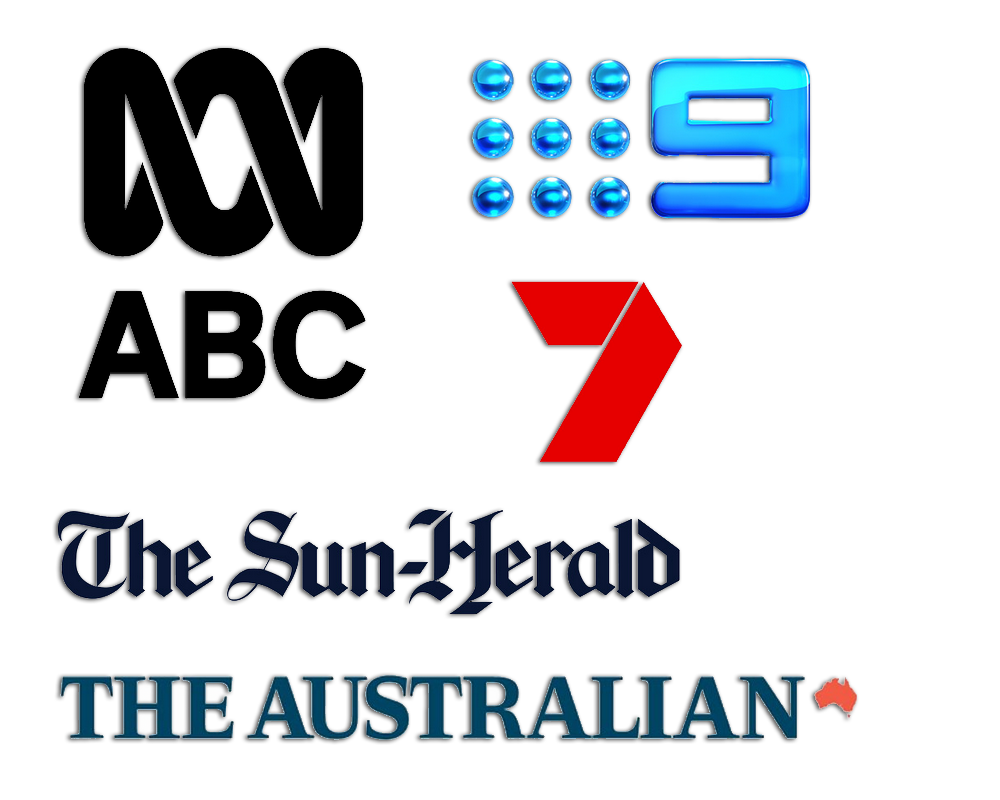This image appears to be a large screenshot taken from the bottom section of a webpage, showcasing its partners and affiliates. At the top of the image, there is a symbol resembling the infinity sign, although it features an extra curve and more angular endpoints, differentiating it from a standard circular arc; this symbol is large and rendered in black.

Adjacent to this symbol is the number nine, presented in a sky blue, metallic two-tone color. Surrounding the number are nine similarly colored blue circles, adding a cohesive design element.

Below these elements, on the left-hand side, the bold black text "ABC" is prominently displayed. To its right is the number seven, portrayed in a striking red color, although its unconventional design still makes it recognizable as a seven.

Further down the image, the text "The Sun Herald" appears in a traditional font style, maintaining a classic and professional look. Lastly, at the bottom, the text "The Australian" is featured, accompanied by an icon depicting the outline of Australia on its right.